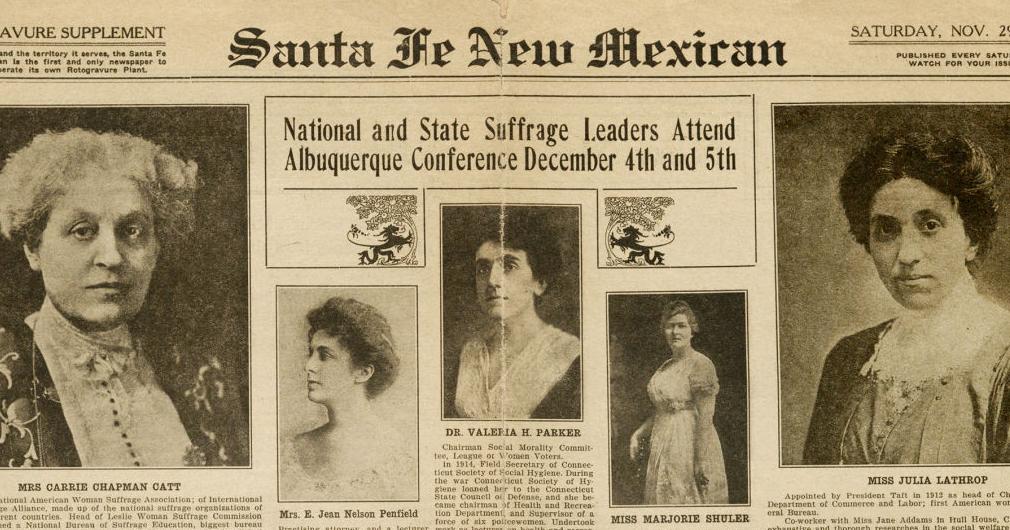The image is a clipping from an old, light brown newspaper titled "The Santa Fe New Mexican." At the top center, it reads "National and State Suffrage Leaders Attend Albuquerque Conference December 4th and 5th." The newspaper appears to have been folded in half at one point, showing a visible crease in the center. The main focus of the article underneath the headline involves portraits of five prominent women leaders from the suffrage movement. From left to right, the women are identified as Miss Carrie Chapman Catt, Mrs. E. Jean Nelson Penfield, Dr. Valeria H. Parker, Miss Marjorie Shuler, and Miss Julia Lathrop. The layout includes two larger portraits on the far left and right, with three smaller portraits aligned in the center. The exact date in November when the newspaper was printed is not fully visible, as it only shows "Saturday Nove" followed by an incomplete "two."